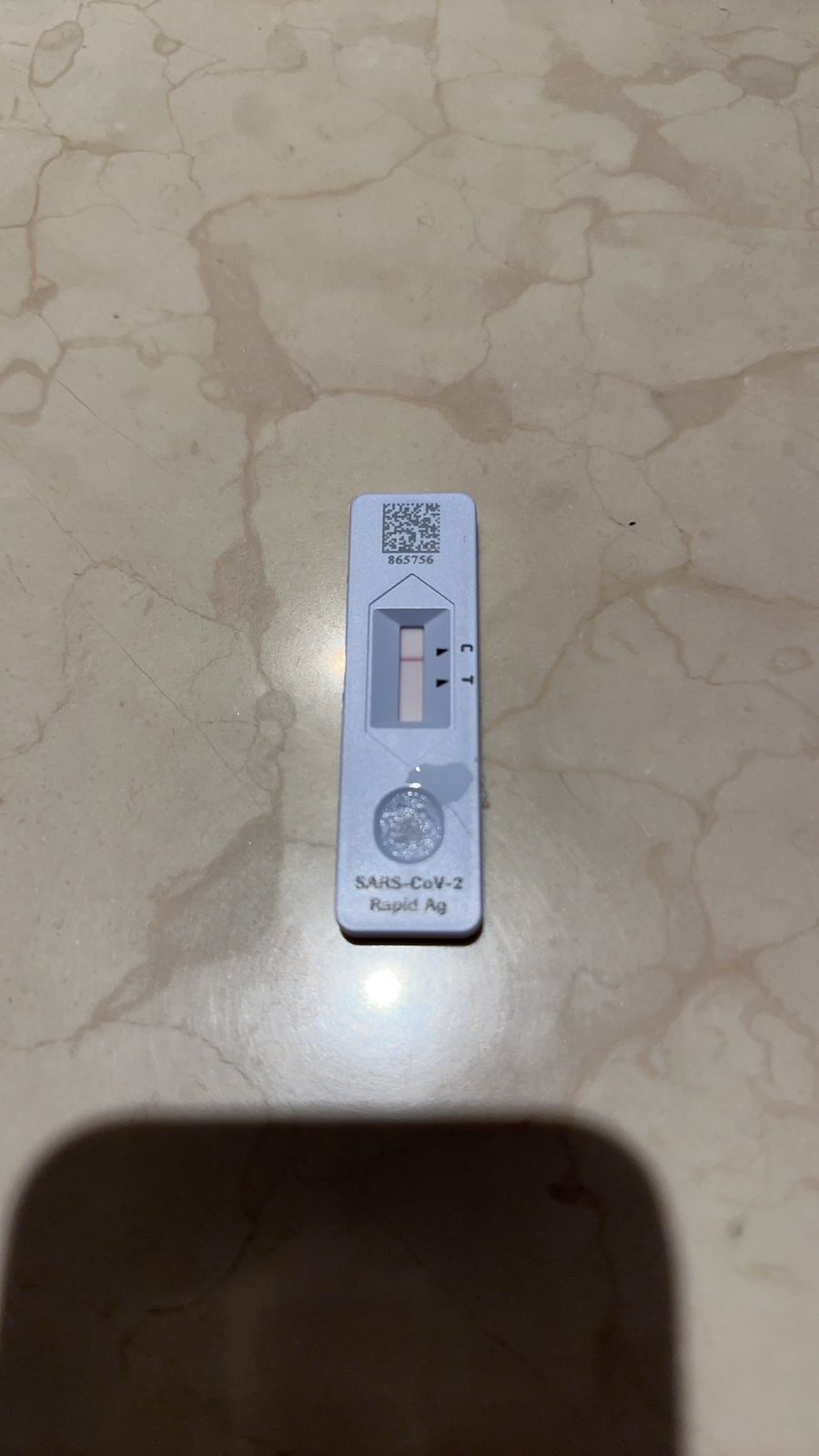The image features a stylish white and cream marble table, prominently showcasing a COVID-19 rapid test. The rectangular, white test device is positioned centrally, with notable details such as a QR code and an identification number "865756" displayed at its top. The test's results area is unique, requiring vertical reading of the "C" and "T" markers rather than the conventional horizontal orientation. Currently, a single faint red line is visible near the "C", indicating a negative result, as a positive test typically displays two lines. Below the result area is a circular well, partially overfilled with the sample, causing a visible splash on the test surface. The bottom part of the test is labeled "SARS-CoV-2 Rapid AG," identifying it as a rapid antigen COVID-19 test. The lower section of the image also captures the shadow of a smartphone, suggesting the photographer likely intended to document the test result, possibly for sharing with friends, family, or perhaps an employer.